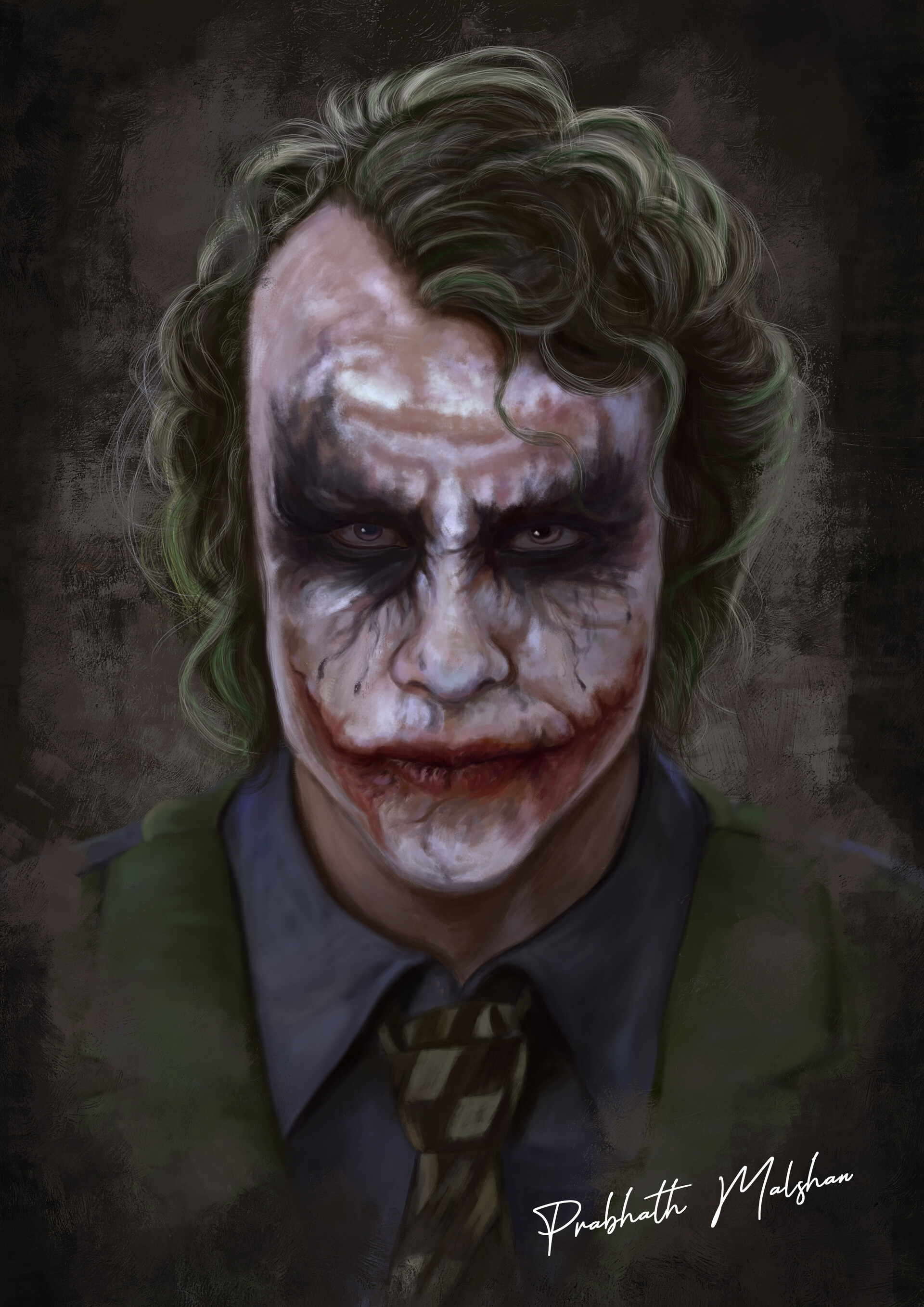This is a detailed artistic depiction of the Joker, inspired by Heath Ledger's portrayal in the Batman films. The artwork features the Joker with a menacing and eerie expression, characterized by a painted white face and black eyes that seem to stare intensely at the viewer. His mouth is exaggerated with red paint, extending to his cheeks in a frown, creating a sinister clown-like appearance. His hair is a mix of green and white, styled in waves that fall down to his shoulders, with some darker highlights giving more depth to the image.

He is dressed in a dark green suit, a navy blue shirt, and a black and beige checkered tie, accentuating his chaotic yet calculated look. The backdrop of the image is a blend of black and gray tones, further enhancing the haunting atmosphere of the portrait. The intricate detailing on the face, hair, and clothing showcases the artist's meticulous attention to realism and texture.

In the bottom right corner of the painting, the artist has signed their name, though it is somewhat difficult to decipher due to the fanciful script. The name appears to be "P-R-A-B-H-A-T-H" followed by a last name starting with "M-A-Y-H-A-N." This signature adds a personal touch, grounding the piece in its artistic origins.